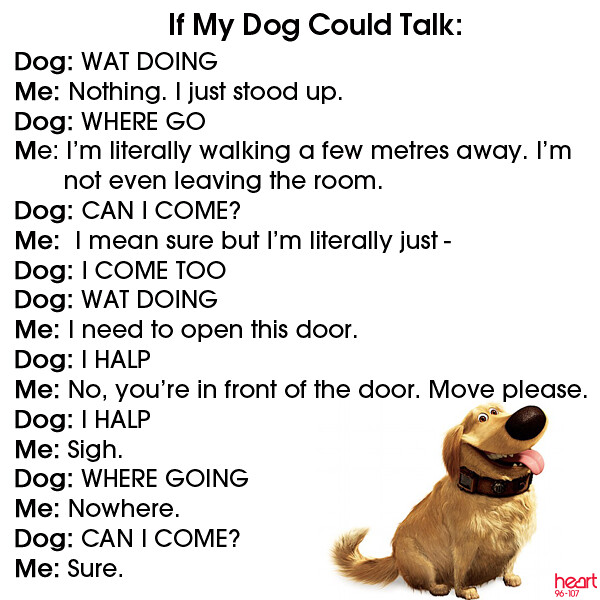The document features a comical portrayal of a conversation between a dog and its owner, titled "If My Dog Could Talk." It is presented on a plain white background with black text. The humorous dialogue captures the dog’s playful and inquisitive nature as it repeatedly asks what the owner is doing and insists on accompanying them, despite the owner’s mundane activities. In the bottom right corner, there is a cheerful, cartoonish depiction of a smiling, bright-eyed brown dog with its tongue out, looking up as if eagerly engaging in the conversation. This visual adds to the comedic effect, imagining the dog talking with its owner and inserting itself into every moment, with phrases like, “Dog: I help,” and the owner’s resigned response, “Me: sigh.”